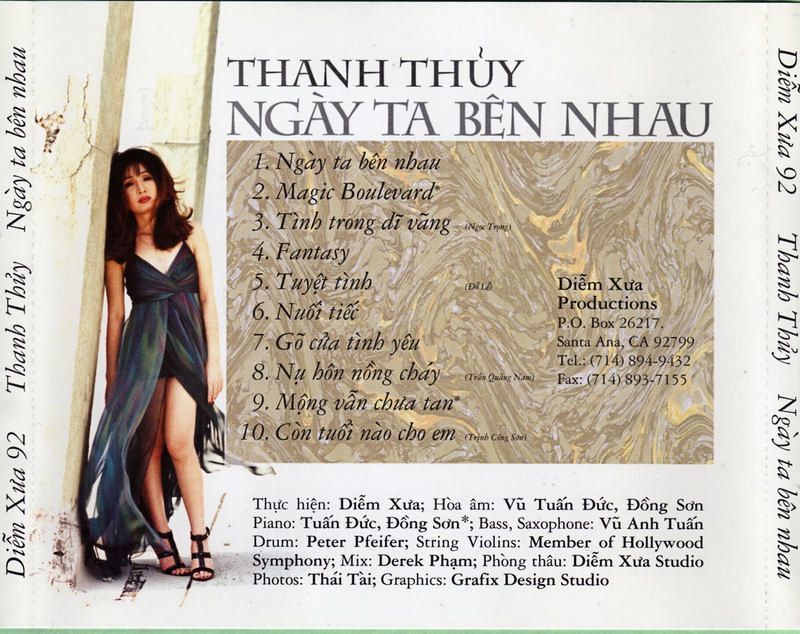This rectangular image appears to be the back cover of a CD or an advertisement for an album. Dominated by a grayish white background, it features a young Asian woman with long black hair, dressed in a stylish bluish-gray dress that is high-cut at the front to reveal her legs. She is leaning to her left against a light tan concrete wall, looking straight ahead with a serious expression. 

Her dress is paired with black, sandal-style high heels. Above her, the text 'T-H-A-N-H T-H-U-Y' is prominently displayed. Below this, in smaller text, is 'N-G-A-Y-T-A-B-E-N-N-H-A-U.' A brown, horizontally swirly rectangle section further down lists ten tracks: 

1. N-G-A-Y-T-A-B-E-N-N-H-A-U 
2. Magic Boulevard 
3. T-I-N-H-T-R-O-N-G-D-I-V-A-N-G 
4. Fantasy 
5. T-U-Y-E-T-T-I-N-H 
6. N-U-O-T-T-I-E-X 
7. G-O-C-U-A-T-I-N-B-Y-E-U 
8. Additional non-English titles 
9. Additional non-English titles 
10. Additional non-English titles 

The bottom part of the image lists musical credits, including 'piano', 'drum', 'symphony', 'bass', 'saxophone', 'string violins', and 'graphics'. The image is bordered by thin dark green lines at the top and bottom, lending it a framed appearance.